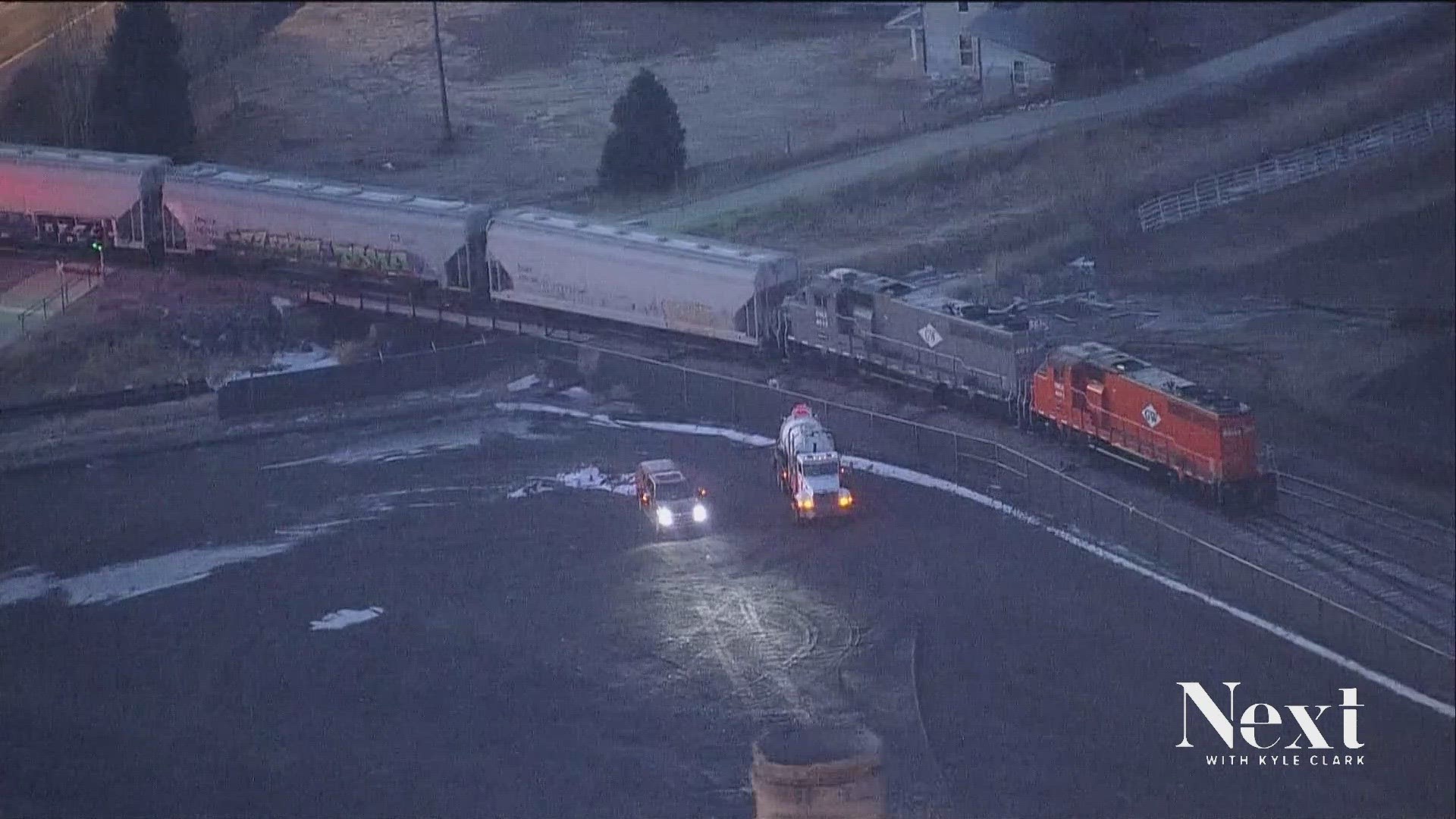The image is a detailed aerial shot taken in landscape orientation at dusk, giving it a dark, gray overtone. The main focus is a train moving diagonally across the frame from the top left to the bottom right. The train compartments are colorful, starting with a red car, followed by a dark gray, then three white cars, and another white car with red accents. Surrounding the train tracks is a chain-link fence, beyond which lies a parking lot featuring a large concrete truck and a station wagon, with a small amount of snow scattered along the fence and grassy edges. Adjacent to the train tracks, there is a field with overgrown grass, a white picket fence, and a two-story farmhouse in the background. In the lower right-hand corner, the words "Next" and "with Kyle Clark" are written in white letters. The landscape is framed by almost black, dark brown, or dark green trees, enriching the scene with a mix of black, white, gray, brown, red, yellow, orange, and green colors.